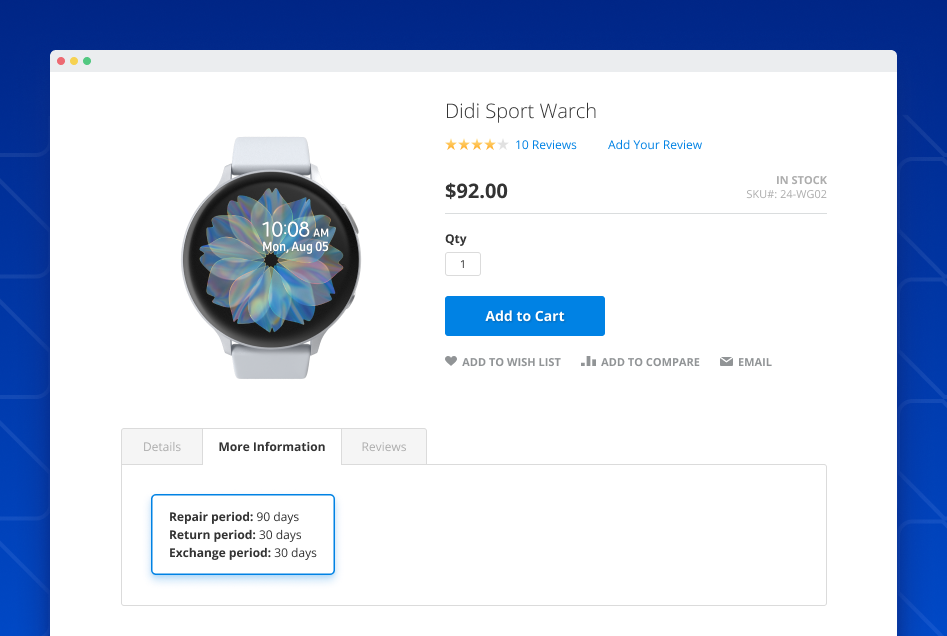Screenshot of a product page from a MacBook or Mac computer displaying a royal blue background with intricate detailing. In the central area of the screen is an image of a product labeled "DD Sports Watch," priced at $92 and currently in stock. The product has a rating of four stars based on ten reviews, and users have the option to add their own reviews via clickable blue links.

Additional options include selecting the quantity (default set to one) and clickable blue links for "Add to Cart," "Add to Wish List," "Add to Compare," and "Email." Below these options are grey-colored buttons labeled "Details," "More Information," and "Reviews," with the "Details" window currently open.

The watch is a white sports model featuring a lotus flower design on the face, displaying the time as 10 a.m. There is also a pop-up box outlined in blue providing information on the repair, return, and exchange periods: 90 days for repairs, 30 days for returns, and 30 days for exchanges.